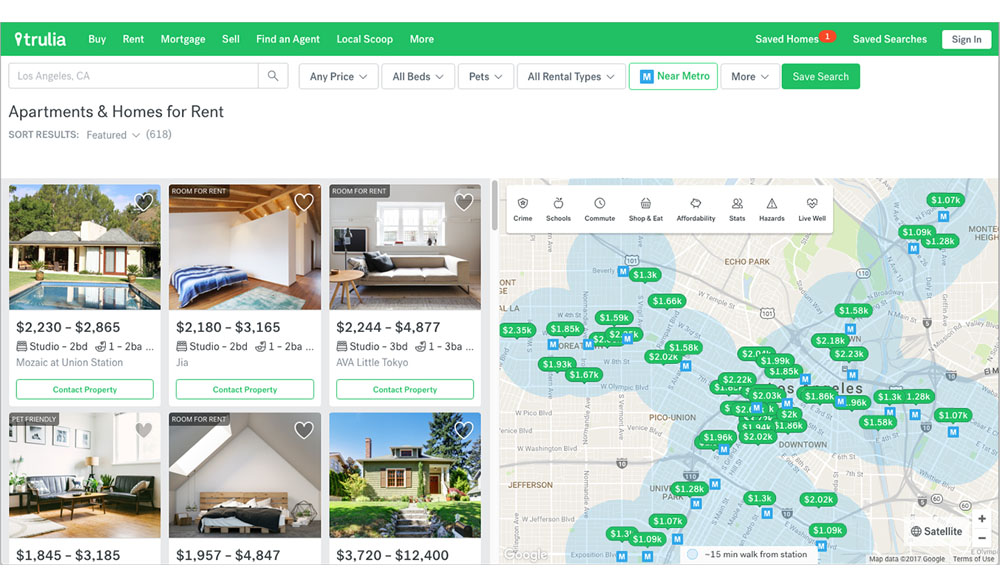This is a detailed description of a horizontally oriented webpage designed for a computer or smart device. The image lacks a distinct background, instead utilizing the white space from the screen itself.

At the top, a long, slim green rectangular navigation bar stretches across the page. In the upper left-hand corner, the bolded word "Trulia" is prominently displayed, followed by less bold options: "Buy," "Rent," "Mortgage," "Sell," "Find an Agent," "Local Scoop," and "More."

On the upper right-hand side, options for "Saved Homes," "Saved Searches," and a "Sign In" button are visible. Adjacent to these elements on the left side, there's a search bar where users can type queries; currently, it reads "Los Angeles, California."

Below the search bar are filter options: "Any Price," "All Beds," "Pets," "All Rental Types," "Near Metro," "More," and a green "Save Searches" button. Continuing on the left side in black text are the words "Apartments and Homes for Rent" and a note indicating that there are 618 featured results.

The primary section of the webpage displays images of various rooms from different houses, showcasing their price range, and the number of bedrooms and bathrooms. To the right of these six images, a dynamic map lists available homes with their prices highlighted in green, clickable for more detailed information.